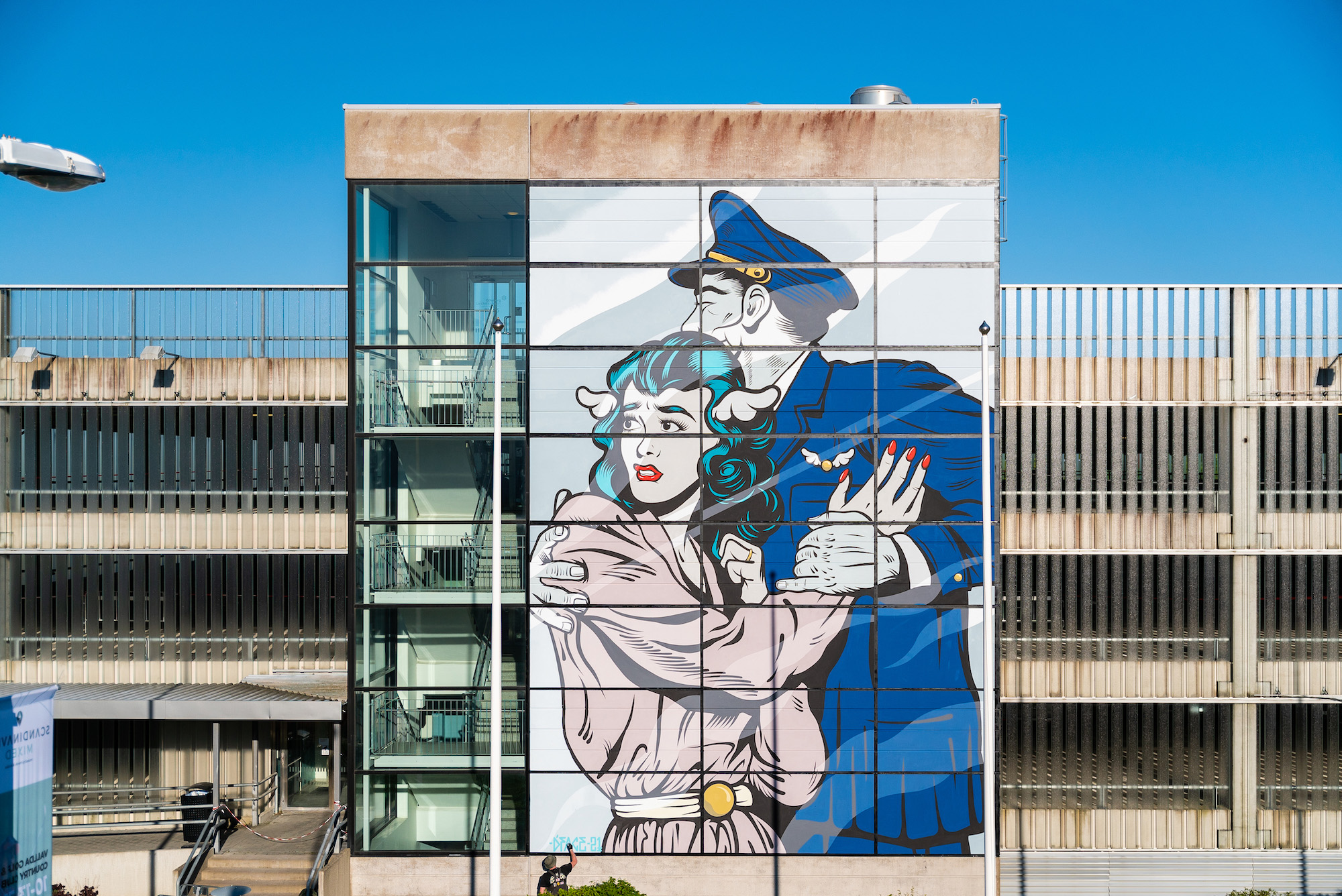The photograph, taken outdoors during the daytime, vividly captures the side of a multi-level parking garage made of cement and featuring tall columns and vertical slats of transparent barrier material. This rectangular image, approximately five to six inches wide and four inches high, showcases a clear blue sky as its backdrop. At the center of the photograph, a large square addition extends from the building, housing the staircases that connect the garage's three visible parking levels and its rooftop.

This extension includes four columns of windows; the first column has transparent glass, allowing visibility into the stairwell, while the remaining three columns feature opaque, white-background windows adorned with a stylized, comic book-like painting. The artwork depicts a scene where a man, dressed as an airline pilot with a blue hat, jacket, and an airplane-wing lapel pin, appears to be protecting a woman with long light-blue hair, a pink outfit, white belt, and red nails. The woman, looking over her right shoulder with a worried expression, contrasts with the man's calm demeanor. Notably, a person is visible at the bottom left of the mural, seemingly in the process of painting a name or signature. The image is clear, well-lit with natural daylight, and provides a highly detailed and colorful representation of the scene.